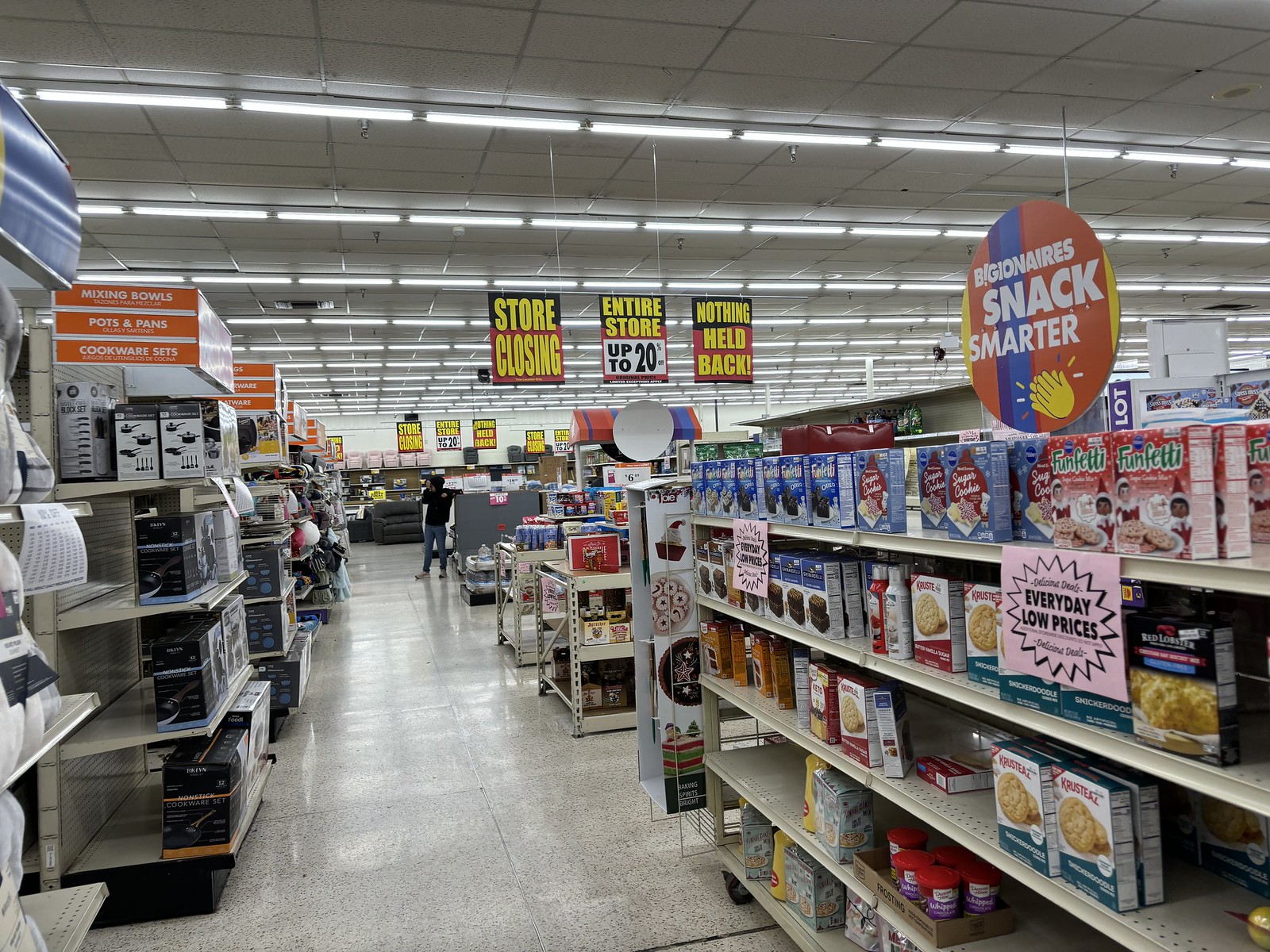In an image showcasing an inexpensive department store that is closing, you can see a tile ceiling adorned with numerous fluorescent lights running horizontally. There are approximately 12 rows of these lights, casting a stark illumination over the store. On the left-hand side, typical gray metal racks with black bases display various kitchen items. Signs labeled "Mixing Bowls," "Pots and Pans," and "Cookware Sets" hang above shelves stocked with corresponding white and black boxes as you move further down the aisle.

To the right, the shelves are filled with grocery items. A variety of baking products like Funfetti, macaroni and cheese boxes, and soup packets can be seen. Further down the aisle, a shorter display catches the eye with a mix of miscellaneous items. In the background, a man dressed in a black shirt and gray pants stands in front of a sofa, drawing attention to the store's mixed inventory.

Prominently hanging from the ceiling in the center are bold signs that announce the store's closure. These signs read "Store Closing," "Entire Store Up to 20% Off," and "Nothing Held Back," all rendered in yellow print on a predominantly red background with black upper sections. The detailed setting captures the essence of a store winding down its operations, with shelves slowly emptying and sales signs signaling the end.